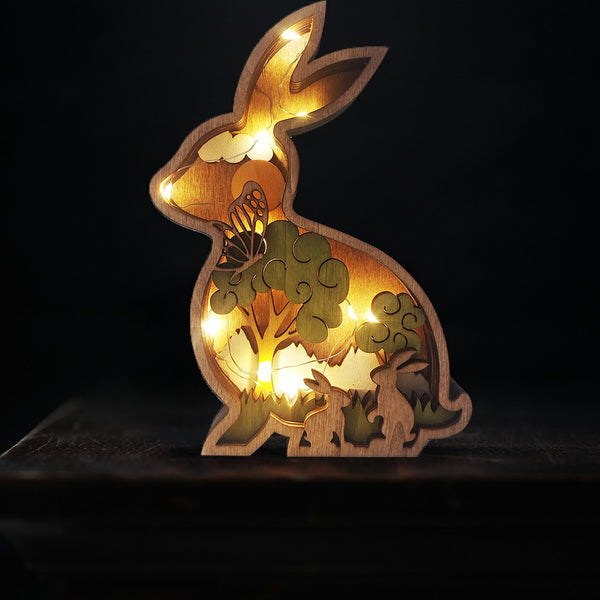A captivating wooden cutout sculpture of a bunny rabbit sits on a dark table against a black background. The rabbit, which appears to be hollowed out, features intricately carved details illuminated by LED lights that transition from white to yellow-orange hues throughout its body. These lights begin at the pointy ears and cascade down to the lower parts, lighting up the entire scene within the rabbit.

Inside the hollow center of the bunny, a detailed tableau unfolds. At the bottom, near its tail, two smaller wooden cutouts of rabbits appear to be engaged in a conversation. One bunny is on its haunches, with its ears sticking out as it looks to the right, while the other stands up on its hind legs, slightly taller than the first. They are positioned in a grassy field flanked on one side by a large tree and on the other by a smaller tree. The background decoration features a possible depiction of white mountain tops in the distance, adding depth to the scene.

Towards the head of the larger rabbit, the inclusion of a wooden butterfly with its delicate lattice wings and dark body adds a whimsical touch. An orange circle, possibly representing the sun, is also carved near the top, adding warmth to the composition. The entire piece is meticulously designed, making it a striking piece of illuminated art that could serve as an enchanting nightlight.